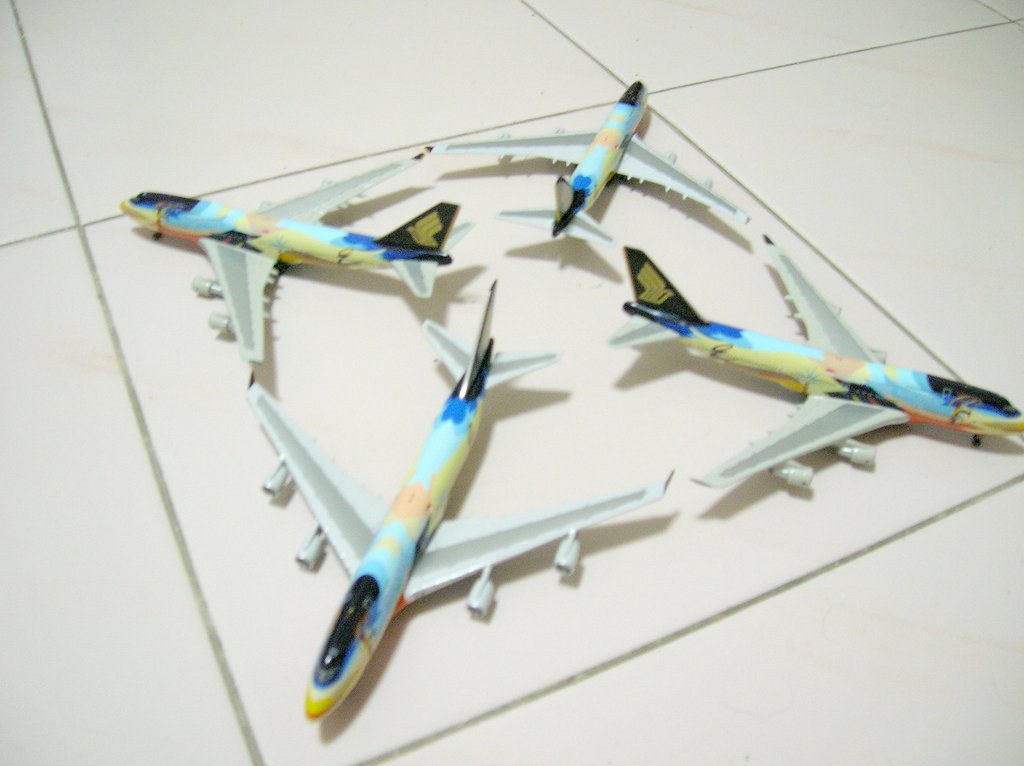This photo depicts a bright indoor setting with a white, cream, and pink-tinted ceramic tile floor, separated by gray mortar lines. At the center of the image, four colorful model airplanes create a symmetrical, star-like formation by aligning their wingtips together. Each airplane's nose points towards a corner of a single large tile.

The model airplanes are intricately detailed: their bodies showcase a blend of pastel colors including blue, pink, and yellow, creating a vibrant swirl across each fuselage. Their cockpits are uniformly black, obscuring any potential windows. These planes also feature gray wings with two jet engines on each, totaling four engines per aircraft. The tails of the planes are black, adorned with a minimalistic gold bird-like symbol.

The light source from above casts soft shadows of the planes onto the tile floor, adding depth to the image. This carefully arranged display highlights the colorful designs and meticulous construction of the model airplanes, capturing a snapshot of playful precision.